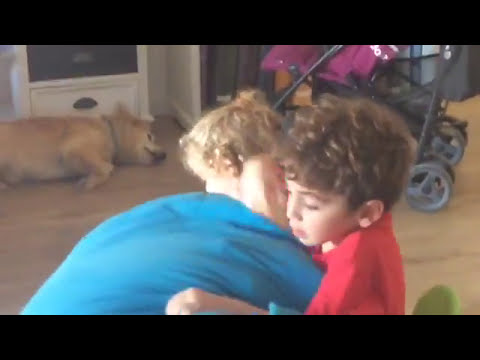In the image, a small boy with curly brown hair, wearing a red t-shirt, is being hugged by a person in a neon blue shirt. The individual's face is indistinct, possibly due to motion blur, making it difficult to determine whether they are an adult or another child. This person appears to have short blonde curly hair. The background features a light-colored wooden floor, a black or gray stroller on the right, and a tan-colored dog sleeping on the floor to the left. The image is also bordered by a thick black edge at the top and bottom.